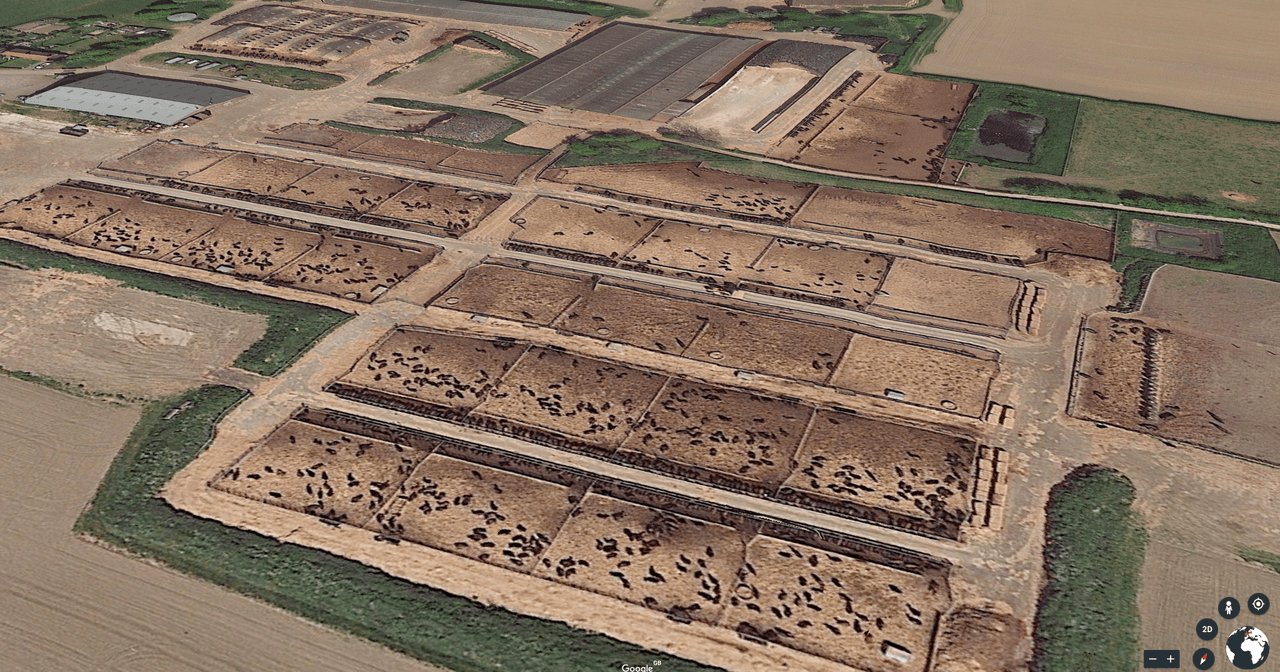This color photograph, taken from a drone, captures an aerial view of a fish hatchery. The landscape is divided into meticulously manicured, rectangular sections, each filled with water where multiple black fish can be seen swimming. Pathways run between these sections, bordered by channels that feed water into the tanks. In the background, several structures are visible, distinguishable by their different colored roofs—some are gray, others tan. Additionally, there are cleared areas of land suggesting future expansions similar to the existing hatchery. On the bottom right of the image, a navigational display features a spinning black globe overlaid with white country shapes, alongside several icons including a navigator, 2D view, walking mode, bullseye, and volume control. The setting also includes a grassy field and a large concrete parking lot, contributing to the realistic and representational style of the photograph.